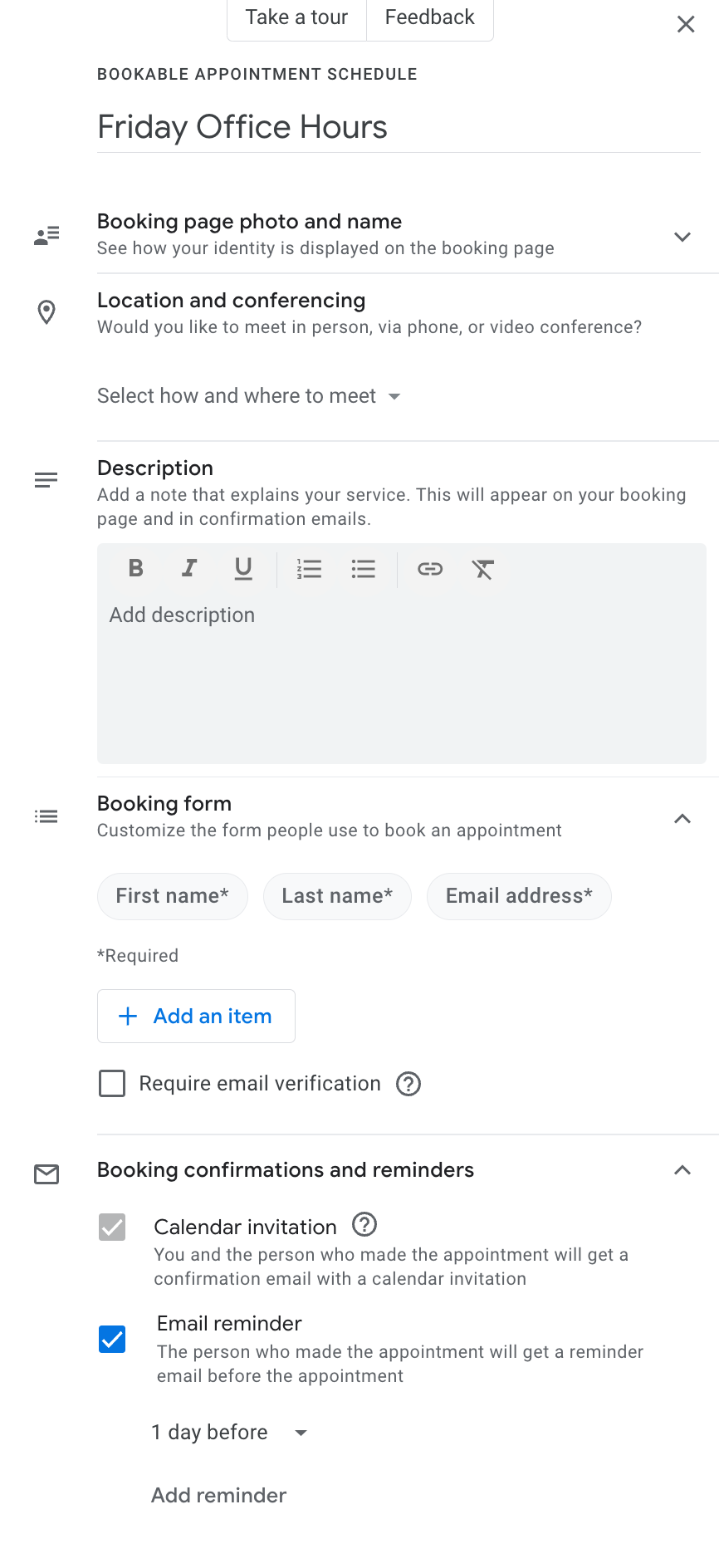At the top of the screen against a white background, bold text reads "Take a Tour and Feedback." Below this, in a slightly heavier font, is the title "Bookable Appointment Schedule - Friday Office Hours." Next, there is a section labeled "Booking Page," which includes a photo and name field with the instruction, "See how your identity is displayed on the booking page." A dropdown menu is available for viewing more information here.

The next section, titled "Location and Conferencing," asks, "Would you like to meet in person, via phone, or video conference?" and provides a dropdown for additional details. 

Moving down, there's a field labeled "Description" prompting the user to "Add a note that explains your service. This will appear on your booking page and in your confirmation emails." A sizable text box follows with options for bold, italics, underline, and other text formatting tools.

Further below is the "Booking Form" section, which instructs users to "Customize the form people use to book an appointment." Required fields include "First Name," "Last Name," and "Email Address," each marked with an asterisk. Users can add additional items via a plus sign or choose to enable an "Email Verification" requirement.

The final section, "Booking Confirmations and Reminders," explains that both the user and the person who made the appointment will receive a confirmation email with a calendar invitation. There's also an "Email Reminder" setting that sends a reminder email to the person who booked the appointment one day before, with a dropdown option to adjust the timing and an option to add additional reminders.